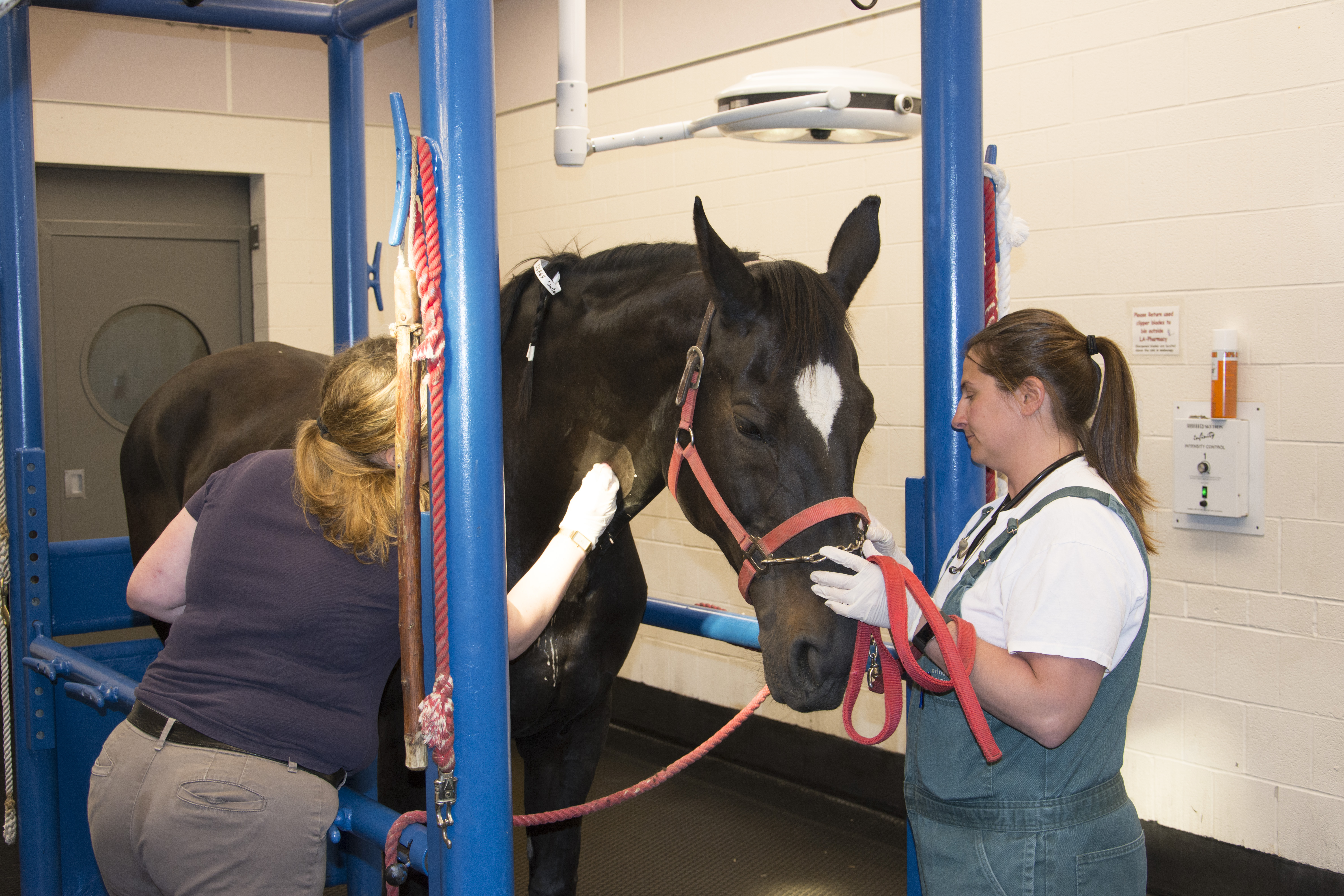In this detailed image, two women are attending to a dark brown horse with a nearly black coat and an upside-down teardrop white patch between its eyes. Both women are wearing white latex gloves, indicating they are in a medical or training facility, likely a veterinary clinic. The horse is secured within a blue pipe enclosure, resembling a shoeing stock, with a red halter and stud chain over its neck, tied to the frame. 

The woman standing in front of the horse, who has medium-length brown hair in a ponytail, is dressed in blue jean-colored overalls and a white t-shirt. She appears to be touching the horse's nose or handling the harness. The other woman, positioned on the left side of the image, is seen from the back. She has dirty blonde hair in a mid-center ponytail, and is wearing a purple shirt, khaki-colored pants, and a brown belt. She has shaved an area on the horse's right neck side and seems to be preparing to administer an injection with what looks like a tissue or cloth in her hand. 

The setting includes a surgical light above the horse, a painted brick wall in the background, and a black-colored door with a circular window on the left side of the room. There is a red lead rope hanging off some hooks and a first aid kit mounted on the wall, further supporting the clinical environment. The floor is black, enhancing the sterile feel of the facility.